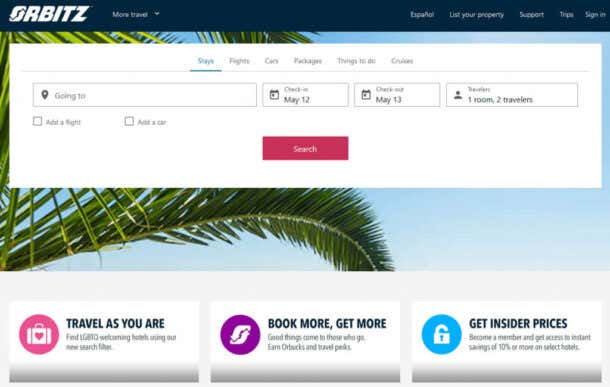This screenshot, captured from a laptop or desktop computer, features the Orbitz website. The top section showcases a prominent blue banner with the Orbitz logo on the upper left—a stylized "O" resembling two arrows in motion. Adjacent to the logo, there are various navigational buttons: "More Travel," "Español," "List Your Property," "Support," "Trips," and "Sign In" situated in the upper right corner.

Just below this banner, a vibrant header image displays the lush green leaves of a palm tree set against an immaculate bright blue sky. Above this image, a comprehensive search window offers various travel options, with buttons for "Stays," "Flights," "Cars," "Packages," "Things to Do," and "Cruises." Users can input details for their destination, check-in time, check-out time, and the number of travelers. Additionally, there are options to add a flight or a car to the search, with a pink "Search" button available to initiate the query.

Further down, the layout includes several informative sections and labels. One notable section is titled "Travel As You Are," promoting LGBTQ-friendly accommodations. Other features highlight the benefits of becoming an Orbitz member: earning Orbucks, gaining travel perks, and accessing insider prices. Membership benefits also include instant savings of 10% or more on select hotels.